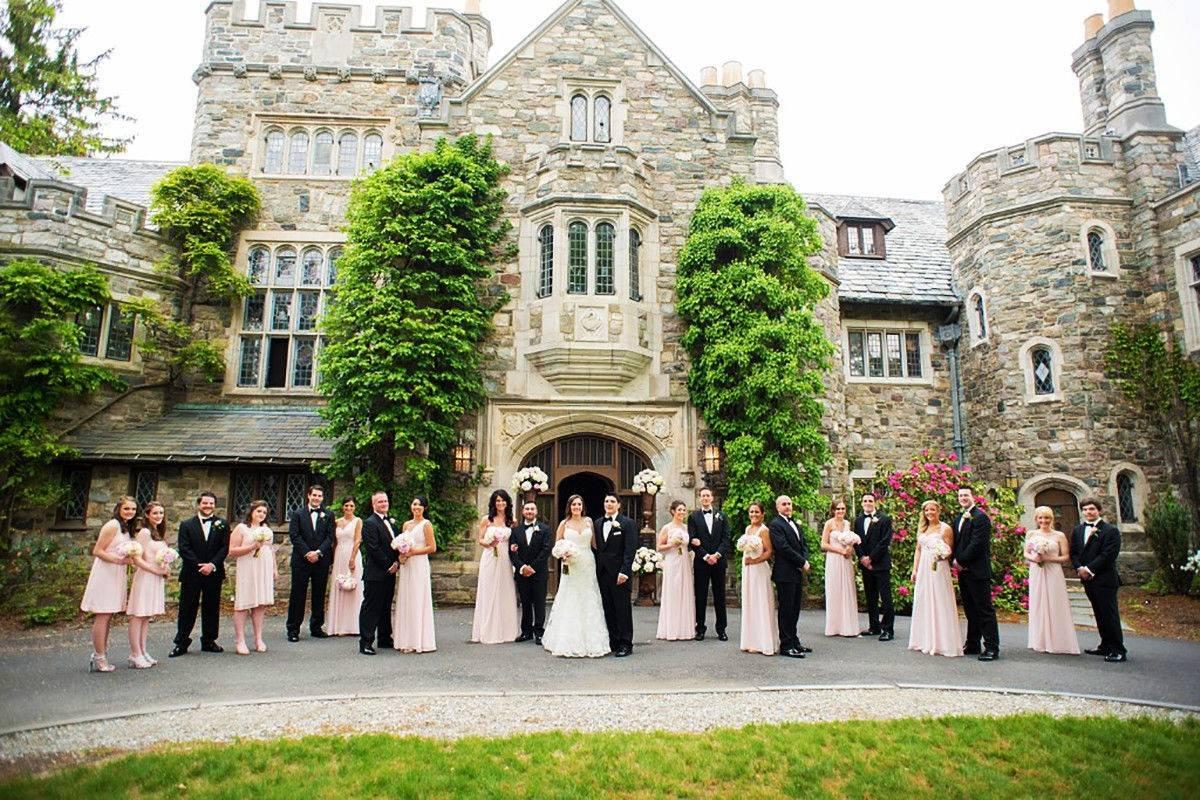In front of a grand, multi-story stone church adorned with numerous pillar sections and an array of windows, a large wedding party gathers for a photograph. The backdrop of weathered stone and intricate architecture provides a timeless and elegant setting. The bride radiates joy in a white gown featuring thin straps and a V-neckline, holding a vibrant bouquet of flowers. Surrounding her are her bridesmaids—two to the left in short, pink dresses, holding flowers and sporting long brown hair, while the remaining bridesmaids wear full-length pink gowns, each with their own colorful bouquets. The groom and his groomsmen stand alongside, all impeccably dressed in black suits, white collared shirts, and black ties. Everyone faces forward, smiling brightly under the clear, sunny sky, embodying a moment of pure celebration and happiness.